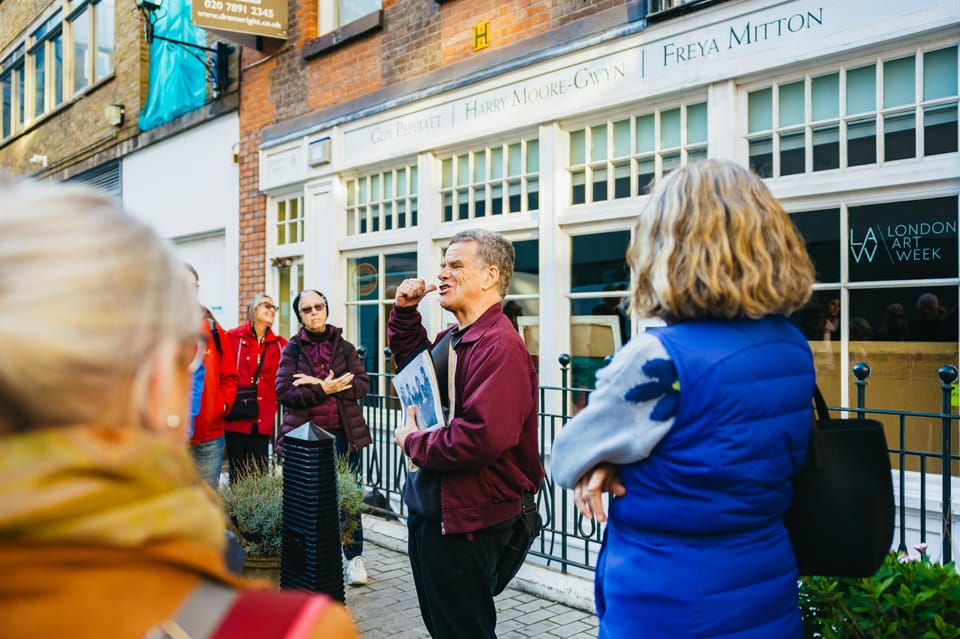In this snapshot photograph, taken on a sunny winter morning, several people are gathered outside a business, which appears to be part of a shopping district in London. The business is housed in a brick building with a blend of red and brown bricks and a front adorned with white-trimmed windows. A sign in a window reads "LA Art Week," and other stenciled names, including "Guy Peirat," "Harry Moore Gwynn," and "Freya Mitton," can be seen.

At the center of the scene is a man in a maroon jacket and dark pants, holding a notebook and pointing back towards the building, seemingly addressing the group around him. The figures around him vary in appearance: one woman in a bright blue vest, another with a pulled-up hairstyle and an orange coat with a scarf, and others in maroon, red, and burgundy jackets. One woman stands with her arms crossed, attentively listening. A small green plant is visible in the bottom right corner of the image. The overall atmosphere suggests a guided tour or discussion related to the London Art Week event, with the morning sunlight casting a bright reflection on the scene.